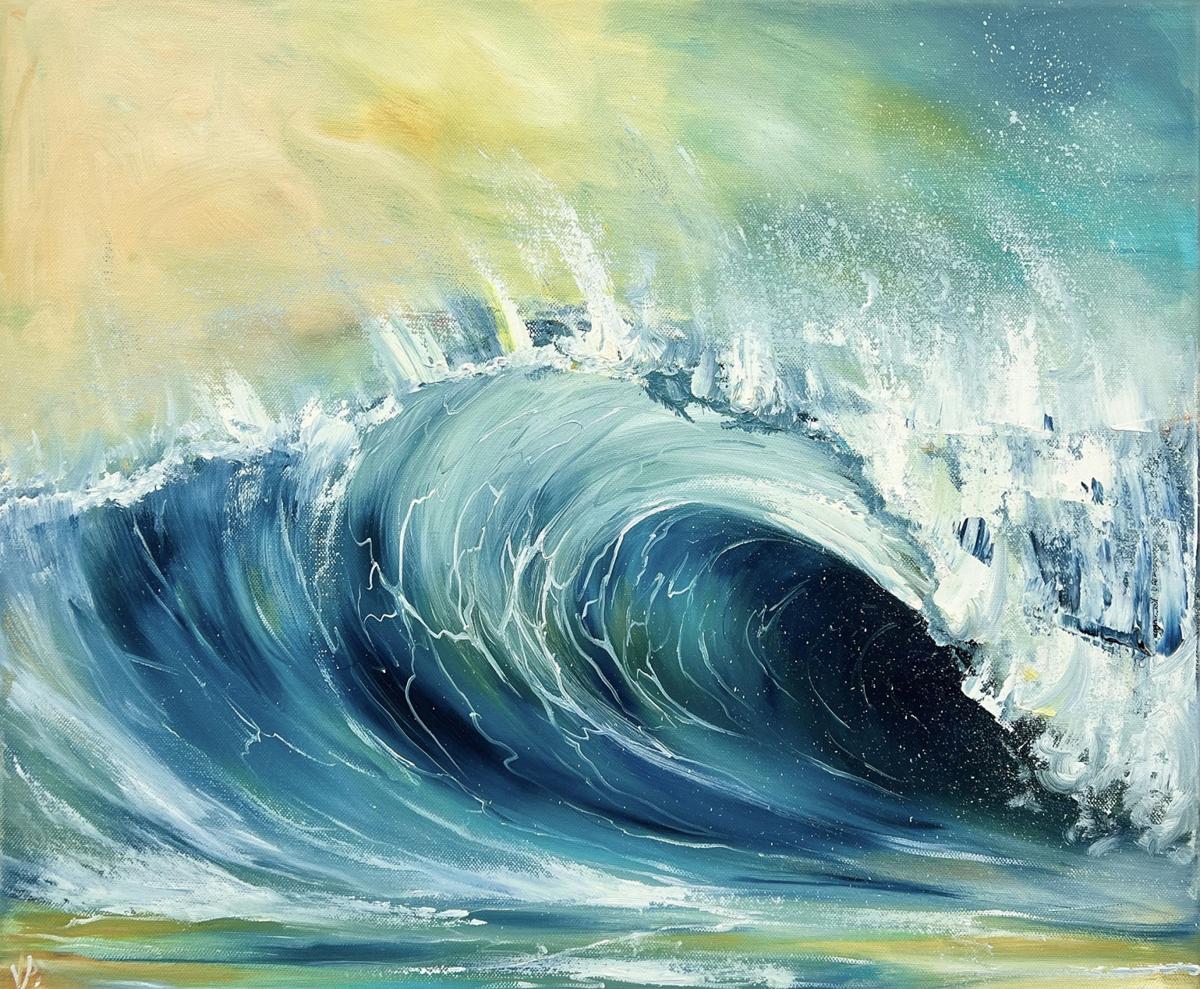The image is a detailed acrylic painting capturing an intense, colorful close-up of an ocean wave, mid-swell, as it begins to crash. The wave curves dramatically, dominating the scene with its aggressive, towering presence, reminiscent of a surfer's tube wave. Splashes and foam are thrown into the air and cascade down, showcasing shades of dark blue, light blue, teal, and green, interwoven with white highlights illustrating the water's ferocity. The backdrop blends a dynamic interplay of yellow and blue hues, perhaps suggesting sunrays piercing through the sky. The left side of the painting transitions from light blue to teal, with a hint of orange, while the right side captures the darker, more tumultuous side of the wave crashing down. The masterful use of color and texture lends a realistic, almost palpable depth to the artwork. The medium appears to be acrylic on canvas, characterized by its rich, naturalistic details.